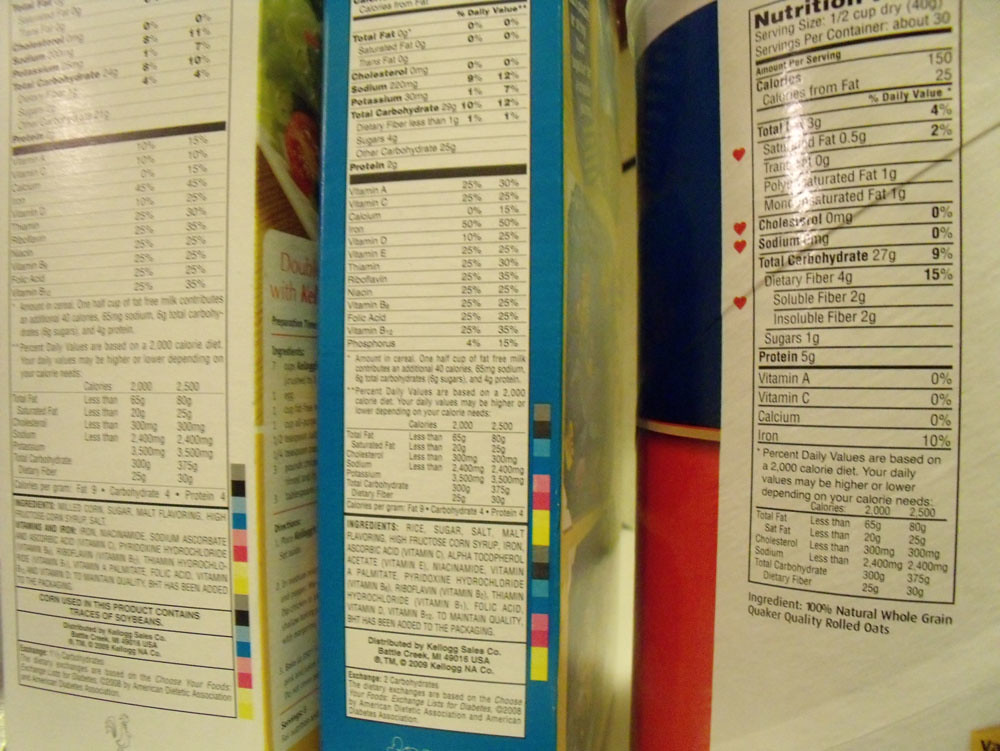The image is a close-up photograph of a breakfast shelf displaying three different cereal boxes. The boxes are arranged side by side, each facing the camera to show their nutritional information panels. 

The box in the center is blue and resembles the packaging of Rice Krispies cereal. The left-most box is less distinct, and its specific brand is unclear from the image. Similarly, the right-most box is not easily identifiable, but behind it is a partially visible can of oatmeal. The oatmeal can features a recognizable design with a blue top and red bottom, hinting at a famous brand with a well-known logo. This meticulous arrangement suggests someone is likely interested in comparing the nutritional content of these breakfast products.